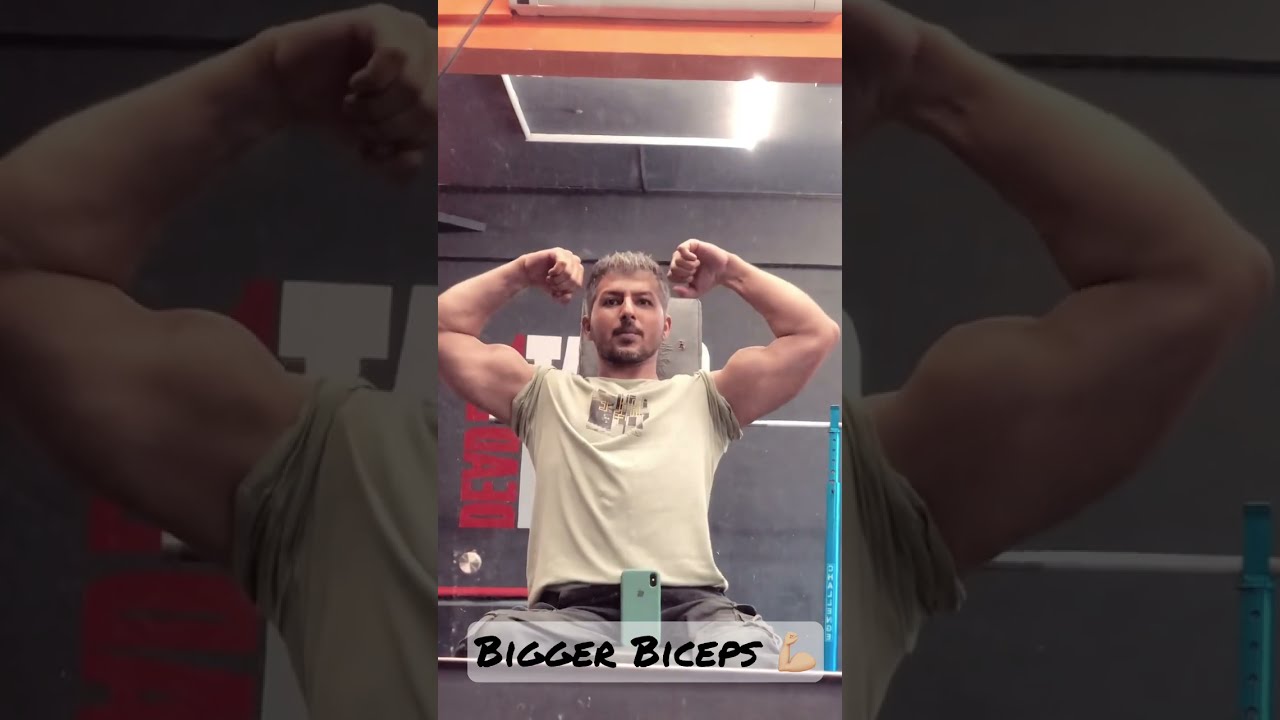The image depicts a muscular Caucasian male sitting in a gym, captured in a unique double-exposure style with two overlapping photographs of the same scene. The prominently visible foreground image shows the man with bleached blonde hair, contrasting dark eyebrows, mustache, and beard. He is wearing a light yellow or green-toned t-shirt with a graphic, and gray pants or shorts. The man is seated on some gym equipment, with his arms raised and fists clenched on either side of his head, emphasizing his well-defined biceps. He appears to be taking a selfie with a smartphone placed between his legs, encased in a teal green cover. Behind him is a gray gym wall adorned with a poster featuring partially legible red and white lettering; the word "dead" is visible but mirrored. The ceiling above includes a bright neon light fixture and an orange bar, contributing to the gym's ambiance. Additionally, a white translucent bar with the words "Bigger Biceps" in hand-printed black lettering is overlayed at the bottom of the image, likely part of the motivational theme of the photograph.